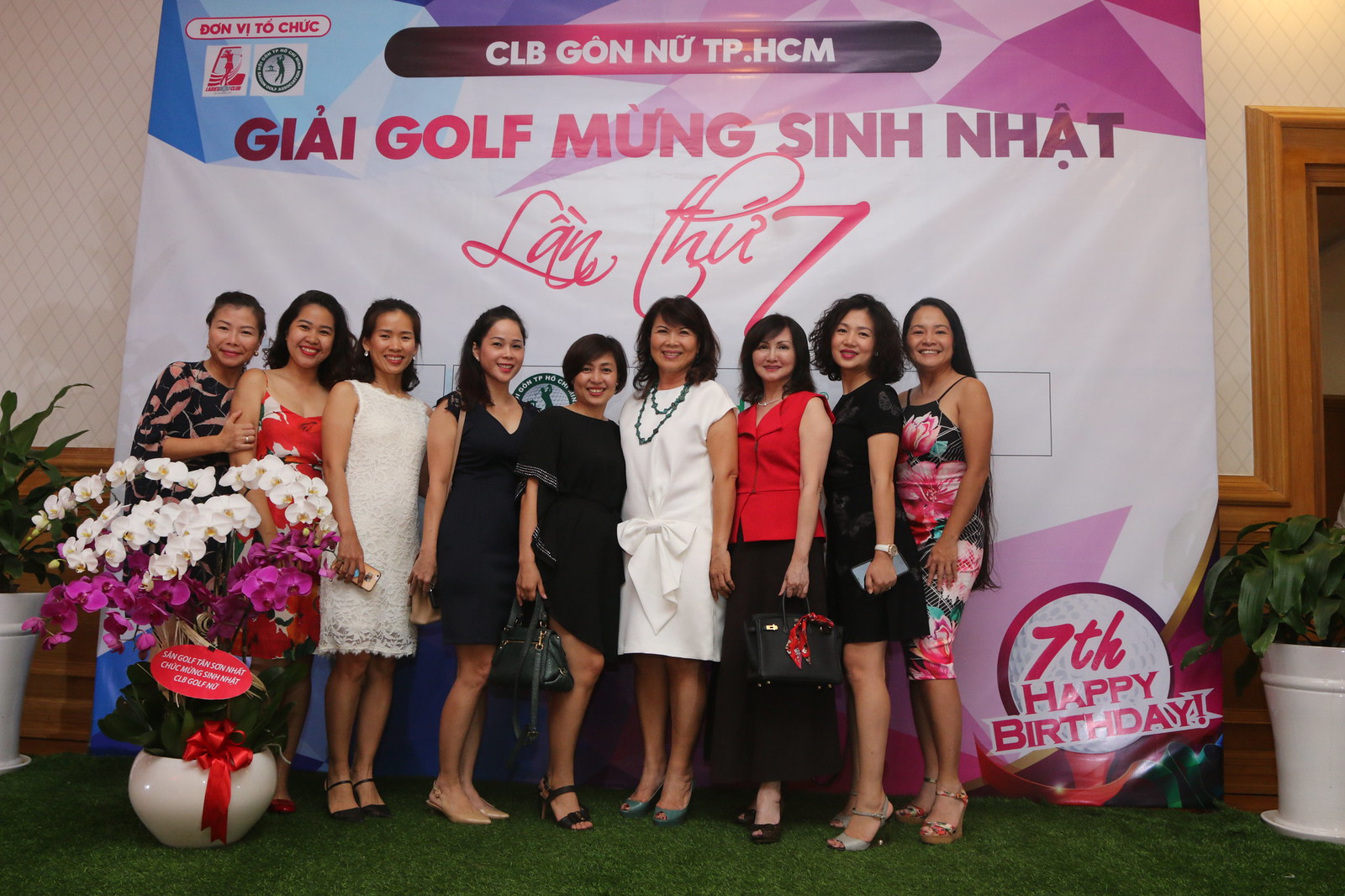In an indoor setting on green carpeting, a group of nine Asian women, dressed in elegant and varied outfits including black, white, and flowery dresses, pose together for a photograph. They are all smiling at the camera in front of a large, eye-catching banner. The banner boasts a vibrant color scheme of blue, white, pink, and purple with geometric shapes and contains text primarily in another language, reading from top to bottom: "GIAI GOLF MUNG SINH NHAT" and "7th Happy Birthday." Beside the women, adding to the scene’s festivity, is a large white vase filled with a beautiful arrangement of white and purple orchids adorned with a red bow and a rubber tree plant.